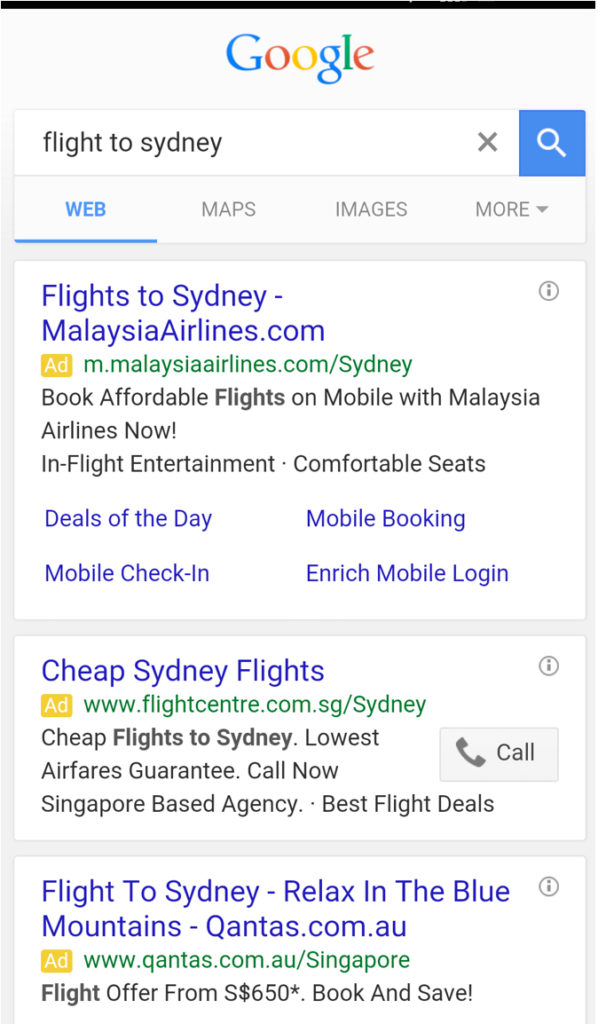The image is a screenshot of a Google search page displaying results for "flight to Sydney." At the top of the search bar, the phrase "flight to Sydney" is clearly visible. 

The first search result is from Malaysia Airlines, with a title reading: "Flights to Sydney | Malaysia Airlines" followed by a link. The description highlights features such as booking affordable flights on mobile, in-flight entertainment, and comfortable seats. It also mentions various services like "day deals of the day," "mobile booking," "Enrich mobile login," and "mobile check-in."

The second search result is from Flight Center, titled "Cheap Sydney Flights | FlightCenter.com." The description promotes cheap flights to Sydney with a lowest airfare guarantee and encourages users to call now. It notes that the agency is based in Singapore and offers the best flight deals.

The third search result comes from Qantas with the title: "Flight to Sydney | Relax in the Blue Mountains | Qantas.com.au." It includes the link followed by "/Singapore" indicating a Singapore-specific offer. The description mentions a flight offer starting from S$650, with an asterisk likely pointing to terms and conditions. It ends with a prompt to "book and save."

Each search result gives potential travelers various options and features to consider for their flight to Sydney.